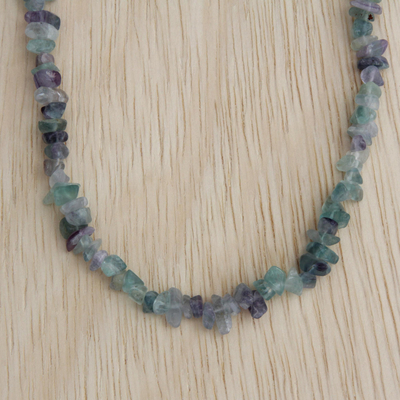The image showcases a necklace laid out on a light brown wooden table with visible grain, characterized by short vertical streaks of darker brown. The table seems to have a slightly whitewashed or pickled finish, giving it an aged yet distinctive look. The necklace forms a U shape and is constructed from several small, irregularly shaped stones and crystals in a variety of blue and green hues. The stones include shades of dark blue, light blue, aqua, baby blue, bluish lavender, and even some near-clear crystals with a bluish tint. The stones are of different sizes, ranging from roughly a quarter-inch to a half-inch, and are slightly translucent, revealing the thread that strings them together. The stones are placed somewhat randomly without a discernible pattern, adding to the overall uniqueness of the piece. Despite the intricate arrangement and diverse color palette of the stones, the overall aesthetic of the necklace and its presentation could be perceived as less attractive.